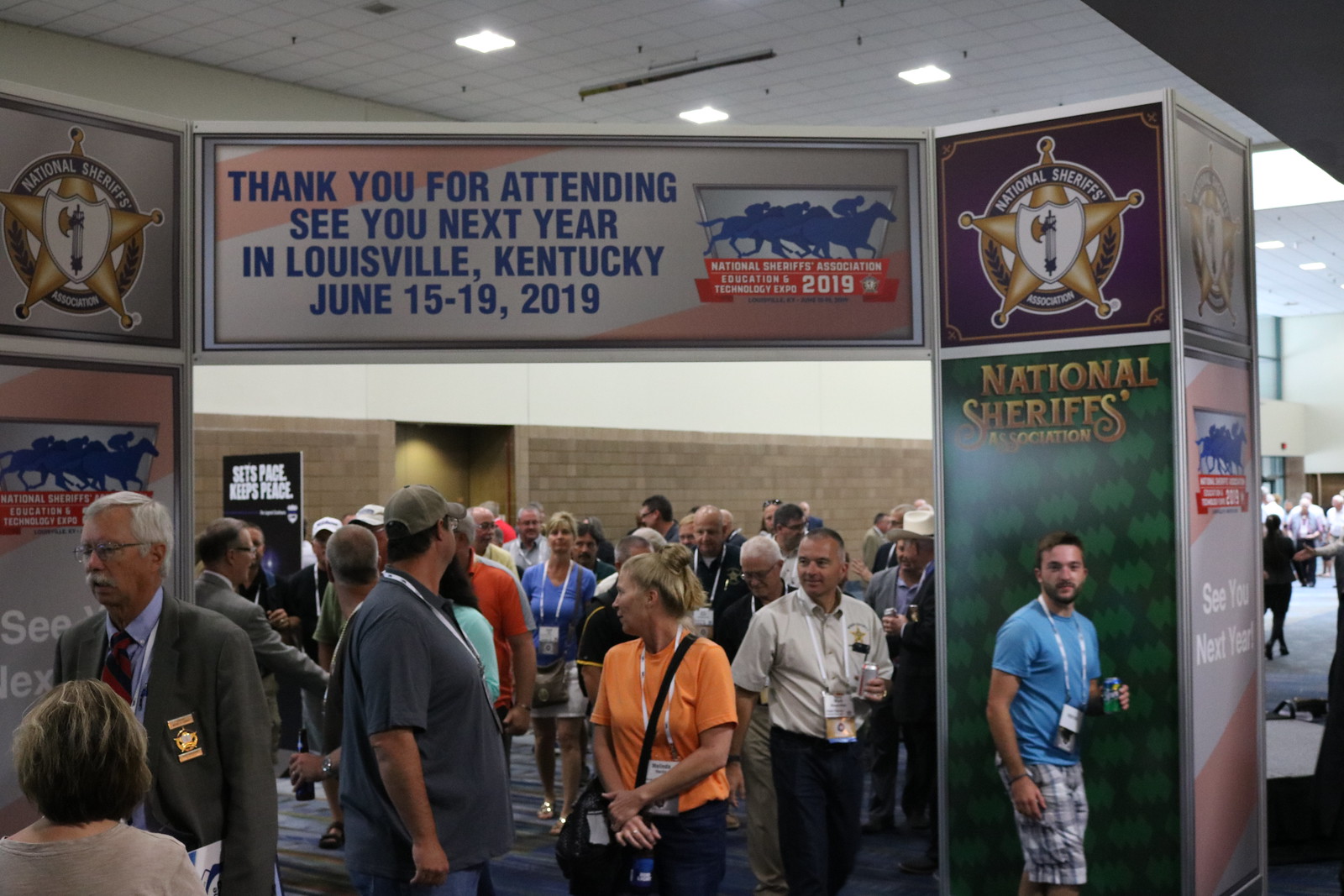This detailed photograph captures the interior of a building bustling with attendees at what seems to be a National Sheriff's Association gathering. Centrally positioned is a lady in an orange t-shirt adorned with a white lanyard, a black strap hanging from her left shoulder to under her arm, and her hands clasped in front of her. Prominently displayed above the crowd is a blue-lettered banner that reads, "Thank you for attending. See you next year in Louisville, Kentucky, June 15-19, 2019," accompanied by a red-titled display beneath it, featuring silhouetted horse riders and the partial text "National Sharks Association, Education 2019."

On both sides of the banner are silver sheriff's badges, each emblazoned with "National Sheriff's Association." The badge on the right is set against a green backdrop with lighter green figures. The scene is illuminated by square ceiling lights casting white light, with a background wall that transitions from brown brick to white halfway up.

The crowd includes a diverse array of individuals, all wearing lanyards with IDs. To the left, a distinguished older man with glasses, gray hair, and a white mustache stands out in a green jacket, burgundy tie, and a badge featuring a gold star. Another noteworthy individual is a man in a light blue short-sleeved shirt and plaid shorts, holding a can and wearing a lanyard around his neck. The atmosphere is vibrant, with many people walking around, creating an engaging and dynamic scene.